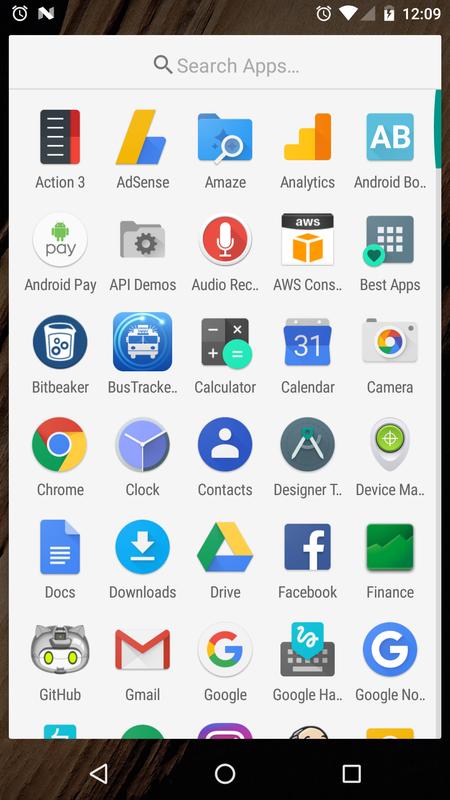The image showcases an iPhone screen displaying the time as 12:09. The battery icon indicates it is approximately three-quarters full, reflecting a decent charge. 

The notification area features an 'N' symbol in gray with a white cross-section and a clock icon. A search bar labeled "Search apps" sits prominently, providing quick access to various applications installed on the phone.

The main screen displays a list of apps, starting with "Action 3," followed by "AdSense," "Amaze," "Analytics," "Android BO," "Enjoyed pay," "API demos," "Audio rack," "AWS cons," "Best Apps," "Bit Break," "Bit Beaker," "Bus Tracker," "Calculator," "Calendar," "Camera," "Chrome," "Clock," "Contacts," "Designer Device," "Docs," "Downloads," "Drive," "Facebook," "Finance," "GitHub," "Gmail," "Google," "Google Ha," and "Google No."

At the bottom of the screen, five partially visible app icons can be seen. Only about a quarter of each icon is shown, making identification difficult. However, the middle icon is recognizable as Instagram with its distinctive purple background designed to look like a person's forehead. The remaining apps feature a blue icon, a green icon, a gold box, and one that resides within a black bar, which also houses standard navigation icons: the home button, the back arrow (triangle pointing left), and a multitasking square.